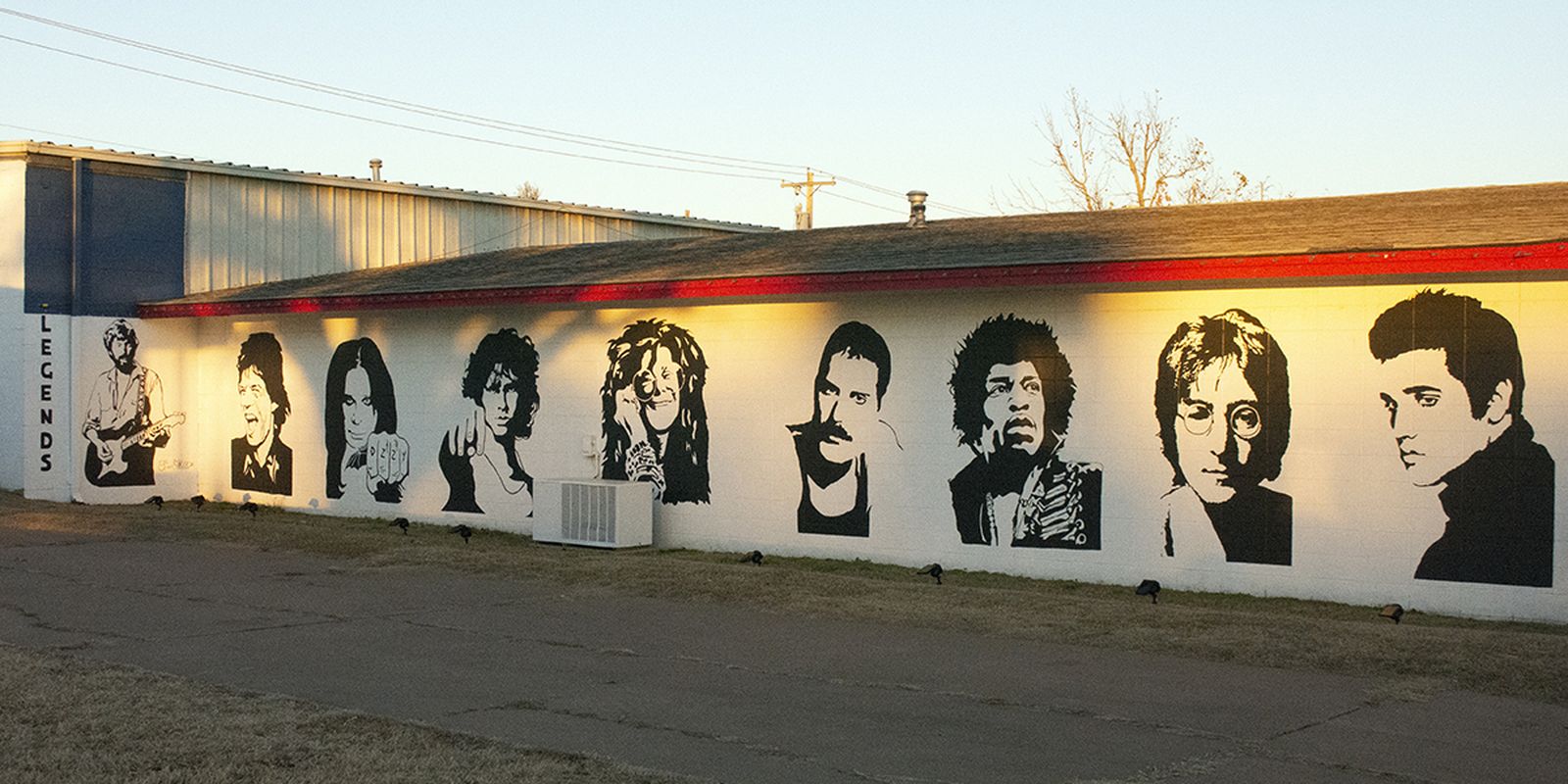This captivating photograph showcases the side of a one-story building, which appears to be a warehouse, featuring a prominent white wall adorned with striking black artwork. The artwork is a series of portraits of iconic American musicians, including Mick Jagger, Ozzy Osbourne, Jim Morrison from The Doors, Freddie Mercury from Queen, Jimi Hendrix, John Lennon from The Beatles, and Elvis Presley. The mural is introduced by the word "LEGENDS" vertically painted on the far left side of the wall. The building has a gray roof with a red trim along the bottom, and an air conditioning unit is visible in front. In the background, one can see another building with white metal siding and a section painted blue, along with a power line and the sparse top of a tree under a light blue sky.